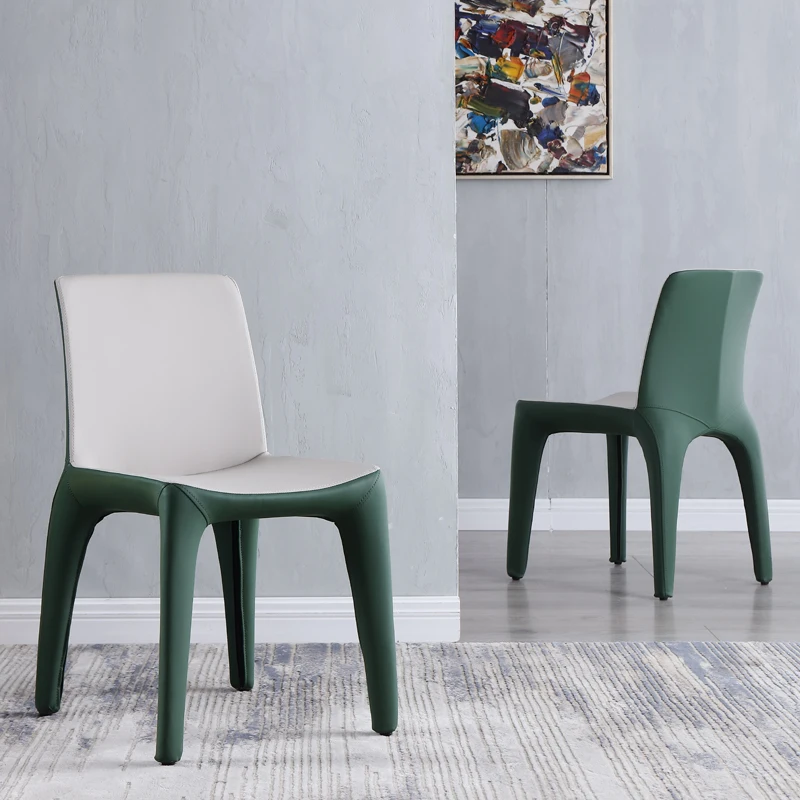The image showcases a room with an art gallery feel, featuring two modern chairs positioned on a white and gray rug that lies on a floor transitioning from wood to carpet. Both chairs have a sleek design characterized by white seats and green legs resembling green leather. The chair on the left is closer to the forefront, while the chair on the right is facing away from the viewer, displaying its green back. The walls are a soft bluish-gray, enhancing the contemporary aesthetic. An abstract painting with hues of yellow, blue, and green hangs above the rear chair, though partially obscured and cropped by the frame of the image. The room is devoid of people, focusing solely on the minimalist, modern furniture and decor.